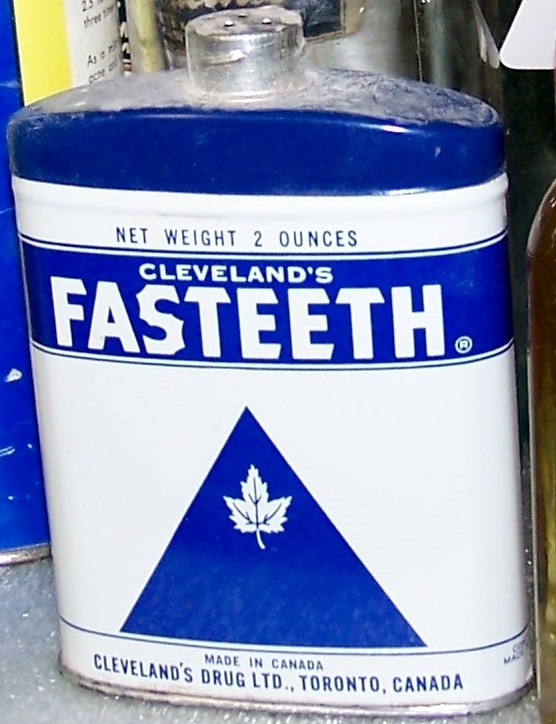This is a vertical close-up image of a metallic canister, designed similarly to a flask with its relatively flat profile and rounded edges. The canister features a seamless blend of blue and white details. At the top, the canister is capped in blue, transitioning into a large white section adorned with various text and designs.

The white portion prominently displays key information. At the top in black text, it reads "Net Weight, 2 Ounces," indicating the product's weight. Below this text, a bold horizontal blue stripe captures attention with the product name, "Cleveland's Fast Teeth," in large block letters, making it unmistakably clear.

Further down, a sizable blue triangle adds a striking visual element. Inside the triangle, at the apex, there is a small icon of a maple leaf, symbolizing the product's Canadian origins. At the very bottom of the canister, additional text details the product's manufacturing information: "Made in Canada, Cleveland's Drug Limited, Toronto, Canada."

Overall, the canister's design is clean and professional, with a distinct color scheme that blends white and blue elements to create an eye-catching and informative packaging.